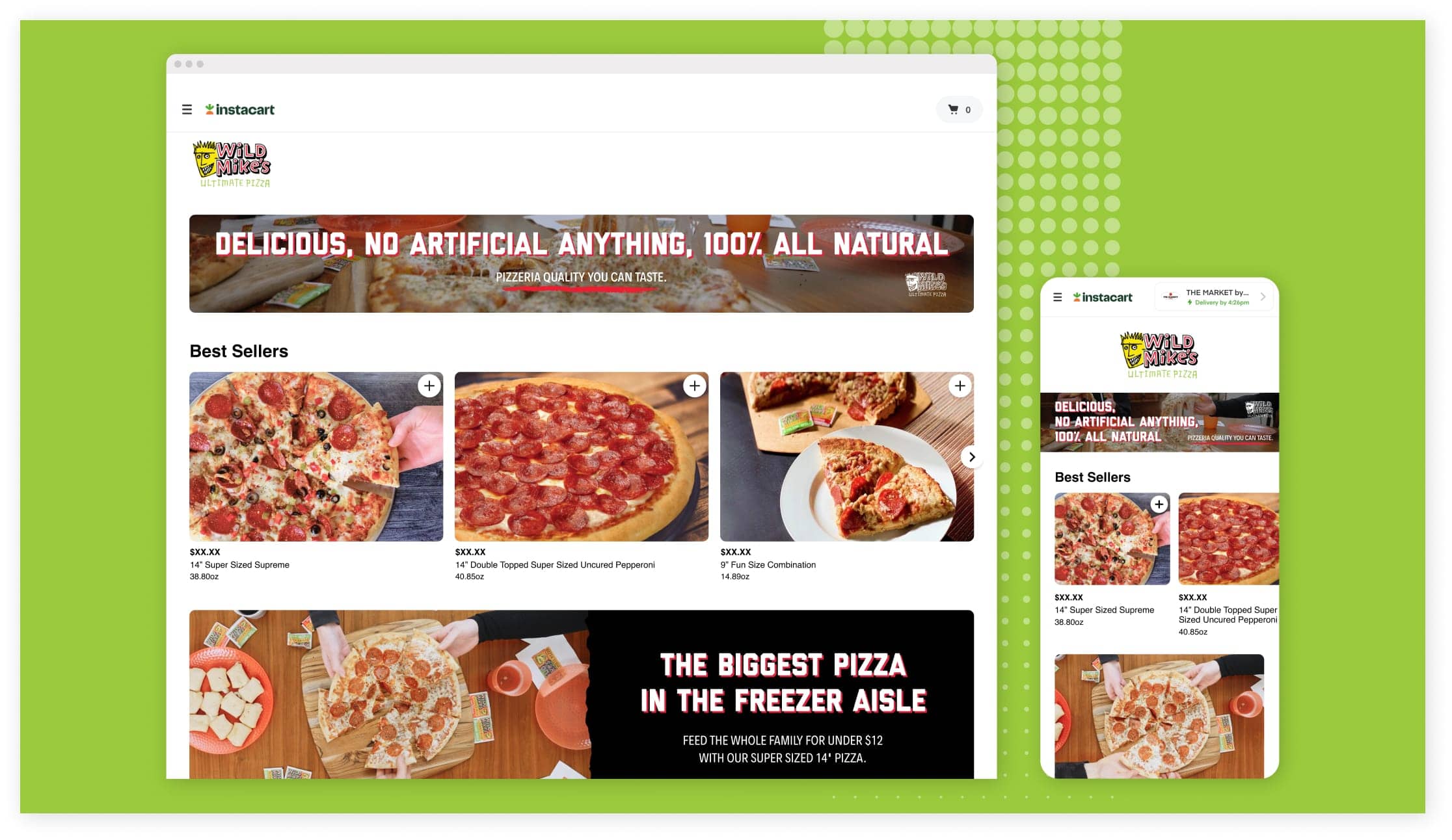The image depicts a promotional advertisement for Texas' Wild Mike's Ultimate Pizza, set against a green background with a grid of dots. The top section of the ad resembles an iMac browser interface, featuring three dots and a hamburger menu. Additionally, there are plus and minus signs, along with the Instacart logo, suggesting easy online shopping. The focal point is the product, Wild Mike's Ultimate Pizza, described as "delicious," "no artificial or anything," and "100% all-natural," with pizzeria quality emphasized by a red underline.

Highlighted in the ad are Texas' Best Sellers, showcasing two types of pizza: "14 Supersize Supreme" and "14 Double Top Supersize Uncured Pepperoni." The ad mentions that Texas boasts "the biggest pizza in the freezer aisle," capable of feeding a whole family of 112 with their supersize 14-inch pizzas. Furthermore, it displays a smartphone indicating the ease of market delivery of pizza by the slice. The ad is visually engaging with a combination of text and images designed to capture the viewer's attention and convey the quality and convenience of the product.